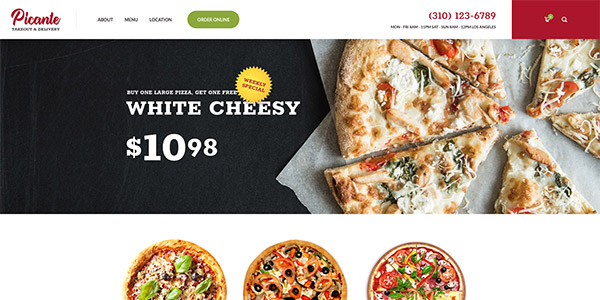Screenshot of the Pecante Website: At the top left of the screenshot, the website's name "Pecante" is displayed in a red, curvy, cursive-like font with the tagline "Takeout and Delivery" directly below it, although the text appears slightly blurry. Immediately beneath the logo, a navigation bar spans the width of the page, featuring four menu options from left to right: About, Menu, Location, and Order Online. The "Order Online" option stands out with white text on a green background.

In the top right corner, a phone number is prominently displayed in red: 310-123-6789. Adjacent to the phone number are the restaurant's operating hours, which indicate different schedules for weekdays (Monday through Friday) and weekends (Saturday and Sunday).

Below the navigation bar, a large advertisement promotes Pecante's weekly special: "White Cheesy Pizza" for $10.98, with a deal to buy one large pizza and get one free. To the right of the promotional text is an image of the White Cheesy Pizza, topped with tomatoes and other fresh vegetables.